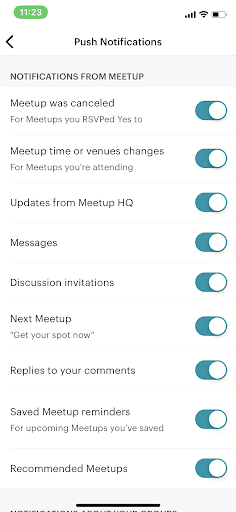A smartphone screen displaying the settings for push notifications in the Meetup app. The time at the top of the screen reads 11:23, flanked by three icons on the left: network status, Wi-Fi signal, and a battery icon, which shows the battery at half capacity. The notification center highlights the settings specifically for push notifications, which are all enabled as indicated by blue slide buttons toggled to the right. Various categories of notifications are listed, including "Meetup was canceled," "Meetup time and venue changes," "Updates from Meetup HQ," and "Discussion invitations." Each category ensures the user stays updated on relevant events and changes within the Meetup app.